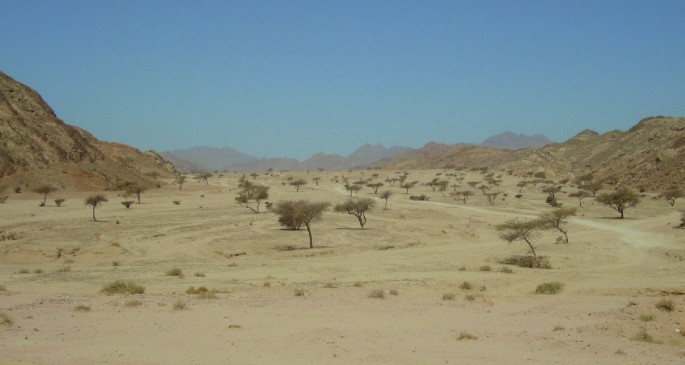This is an outdoor photograph capturing a desert plains area during the daytime. The photo, approximately four to five inches wide and three inches high, showcases a landscape dominated by light brown dirt and sand. Small stumps, mounds of grass, and stunted little trees with thin, dark brown trunks and flat-topped light greenish-brown foliage are scattered across the terrain. Hard-packed dirt and raised rocky hills frame the lower left and right-hand corners, respectively, while a small roadway or path extends from the right side toward the center, meandering through the sparse vegetation. The background reveals brown and gray mountain ranges under a clear, light blue sky, which appears a bit hazy, causing the distant mountains to look fuzzy and obscured. The scene is bisected by faint trails likely made by animals or vehicles, giving the impression of intersecting roads leading toward the mountains on the horizon.